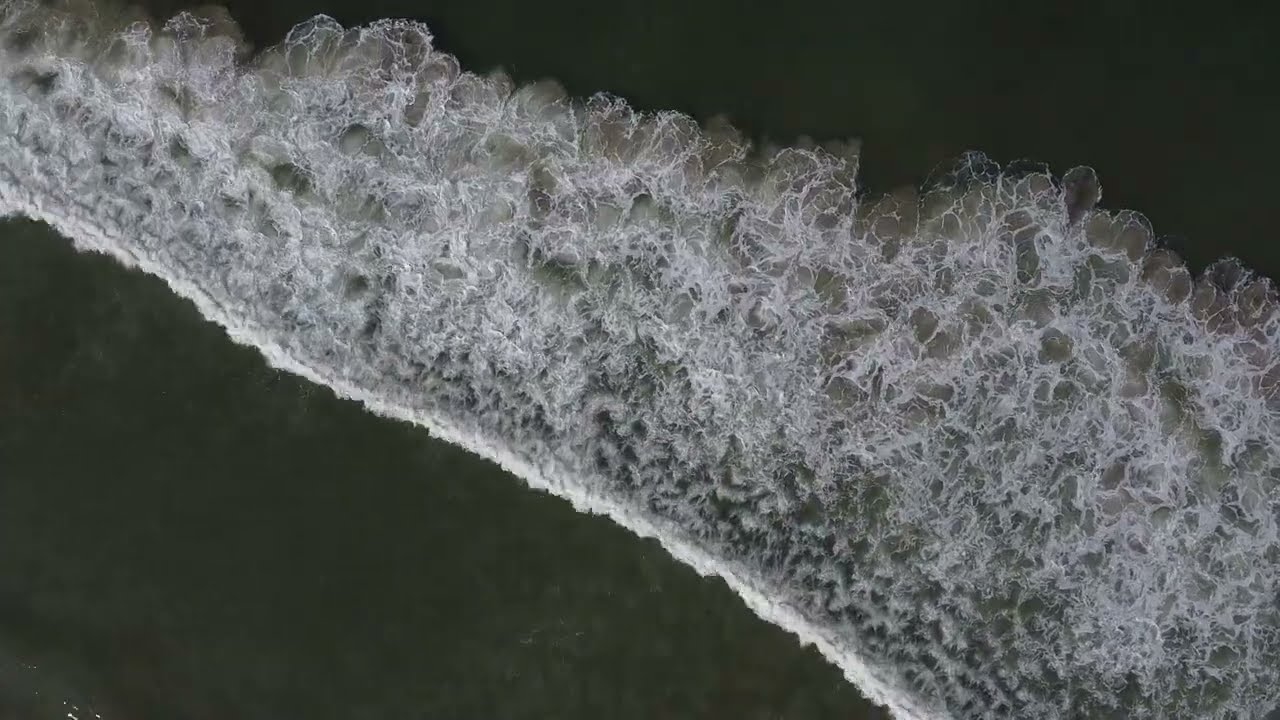This rectangular overhead photograph captures an intriguing scene of a body of water from a bird's eye view. In the top left and top right corners, as well as the bottom left, the water appears calm with a dark greenish-gray hue, suggesting deeper, more tranquil areas. Diagonally bisecting the image from the upper left to the bottom right, there is a striking band of turbulent white water. This foamy turbulence appears as a solid line of a small wave, likely in the back stage before crashing, moving toward an unseen shoreline. Underneath this frothy area, hints of tan coloration suggest the presence of a submerged land bar or rocks. The interaction between the water and these underwater structures possibly creates the noticeable white turbulence, indicating crashing waves that appear to be breaking over shallower areas. The juxtaposition of the calm sections and the dynamic central band of moving water forms a compelling visual contrast in the image.